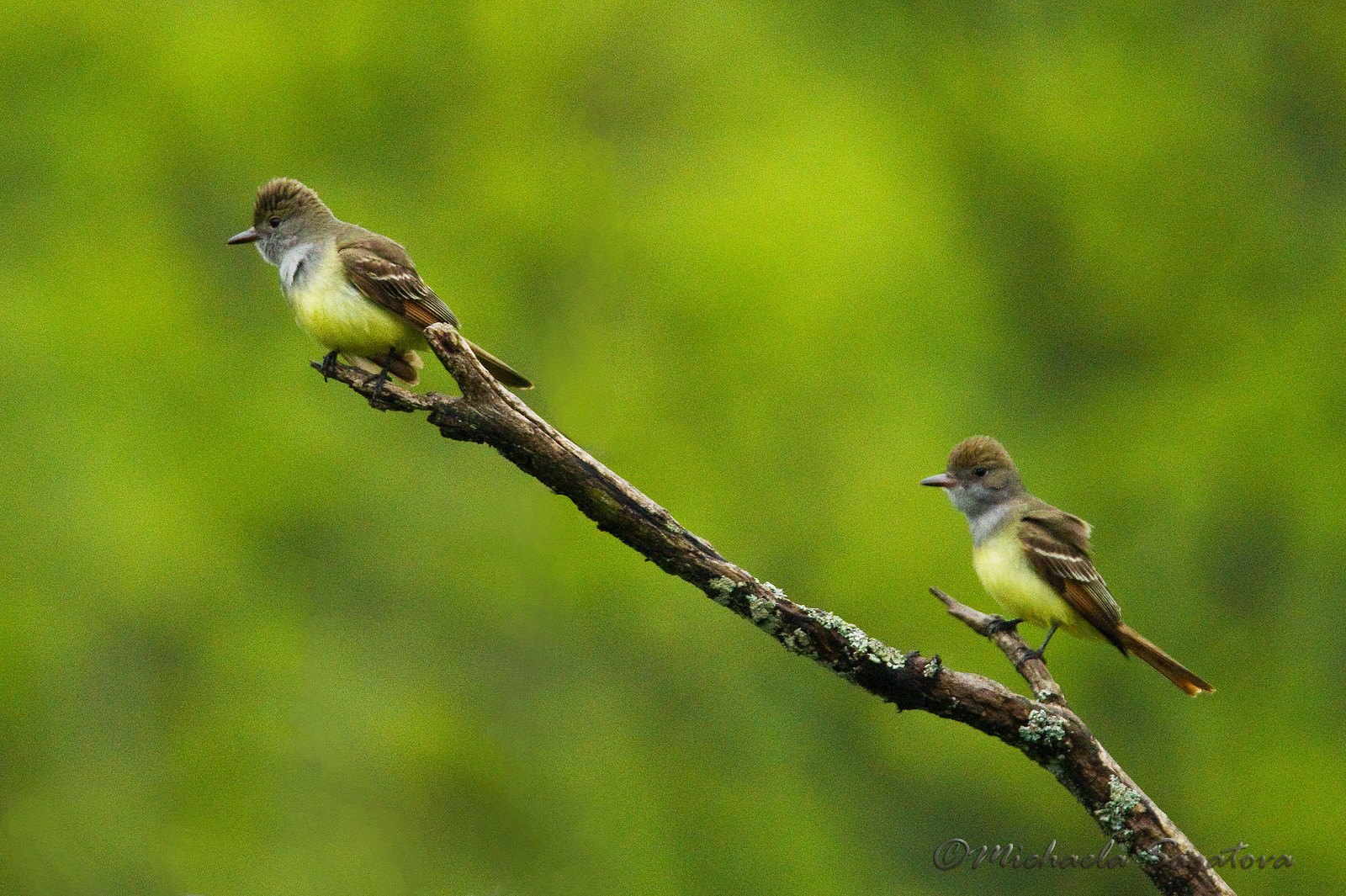The photograph features two similarly colored birds perched on a two-pronged tree branch against a backdrop of blurred greenery. The main branch begins at the bottom right of the image, extending diagonally upwards to the middle-left, where one bird is perched at the tip. This bird has a brown body, a black beak, a yellowish belly, and a head marked with white and black patterns. Facing left, its feathers are fluffed up, and its black eyes are clearly visible. The second bird sits on a small protrusion off the main branch in the bottom right of the image, bearing the same color pattern as the first bird with a dark red beak. Both birds exhibit brown feathers on their wings and heads and appear alert, looking in the same direction. The background is a blur of green, indicative of a dense, leafy environment, and there's an indistinct writing in the bottom right-hand corner that looks like it might be a signature or name. The branch is adorned with patches of lichen, adding to the naturalistic setting.